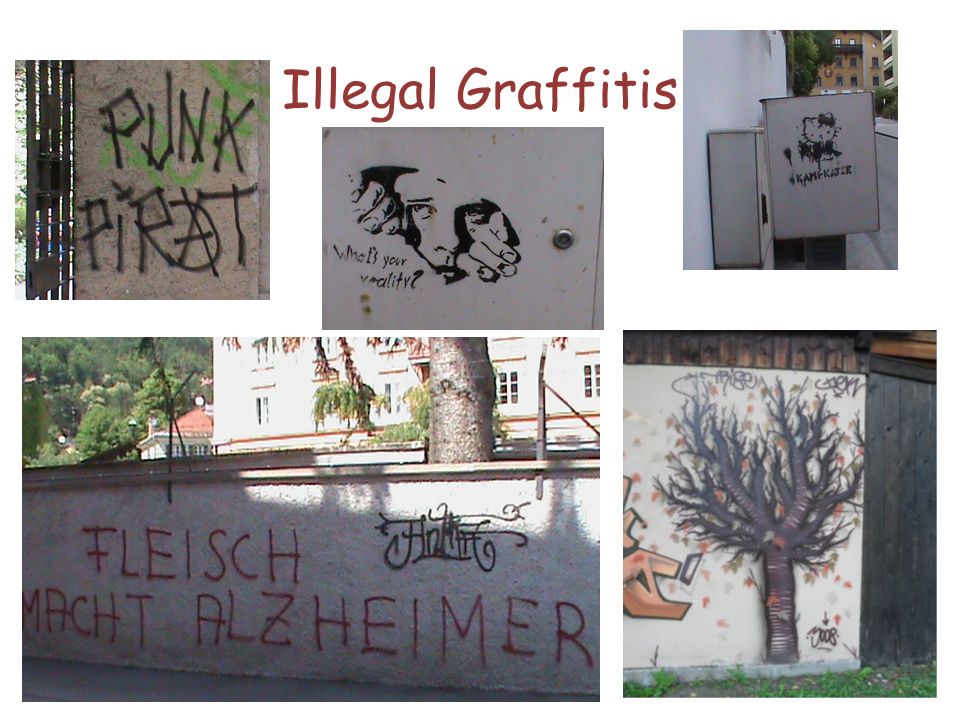The image titled "Illegal Graffitis" showcases a compilation of five distinct pieces of graffiti. The top left graffiti reads "Punk Pirate" in black, accentuated with green lines on the word "Punk." In the top middle, a lifelike depiction of a human face peers out while opening a gap with its arms, with the phrase "Watch Your Vitality" inscribed to its left. Adjacent to this, on the top right, a small Hello Kitty character is painted on a white surface. The bottom left graffiti, spray-painted in bold letters on a wall, reads "FLEISCH, MACHT, ALZHEIMER." Finally, the bottom right features a tree with a few leaves, drawn in purple on a white wall. This presentation spans across a variety of colors including black, green, red, orange, purple, and white, emphasizing the diverse styles and messages of illegal street art.